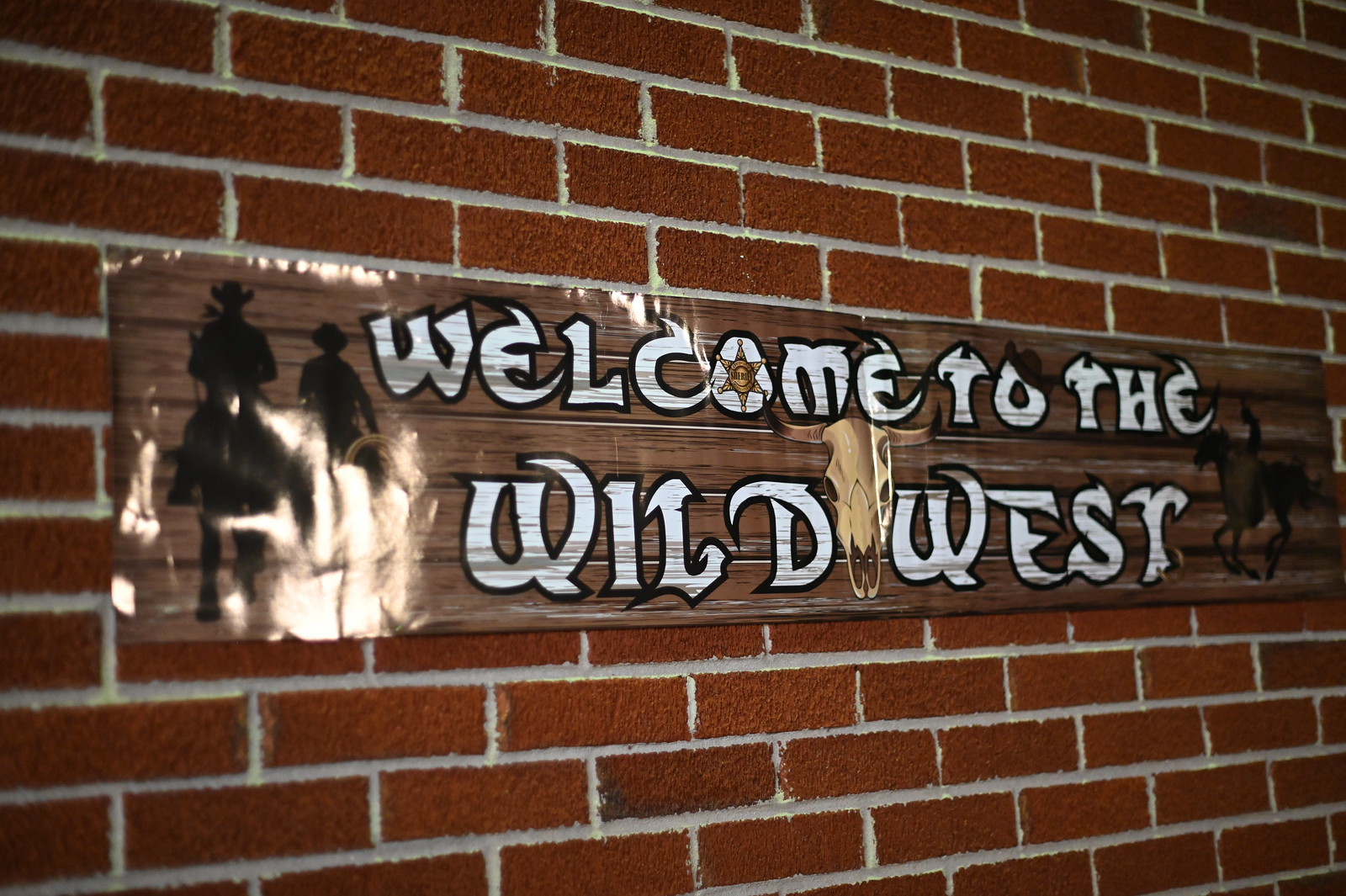This is a rectangular photograph, approximately six inches wide and four inches tall, depicting a reddish-brown brick wall with narrow, long rectangular bricks and white grout. Centrally located on this wall is a glossy, paper banner designed to look like wooden boards, featuring a prominent wood grain pattern. The banner reads "Welcome to the Wild West" in large white letters framed by a black border. The letter "O" in "Welcome" is creatively designed as a sheriff's star. On the left side of the banner, there are silhouettes of two cowboys in black, their hats distinctly highlighting their cowboy style. On the far right, a dark brown silhouette of a galloping horse with a rider, possibly an iconic figure, is depicted, moving towards the left. Additionally, between the words "Wild" and "West," a cow skull is centrally placed, enhancing the Wild West theme. The banner's glossy plastic cover gives it a shiny appearance, making it stand out against the textured brick background.